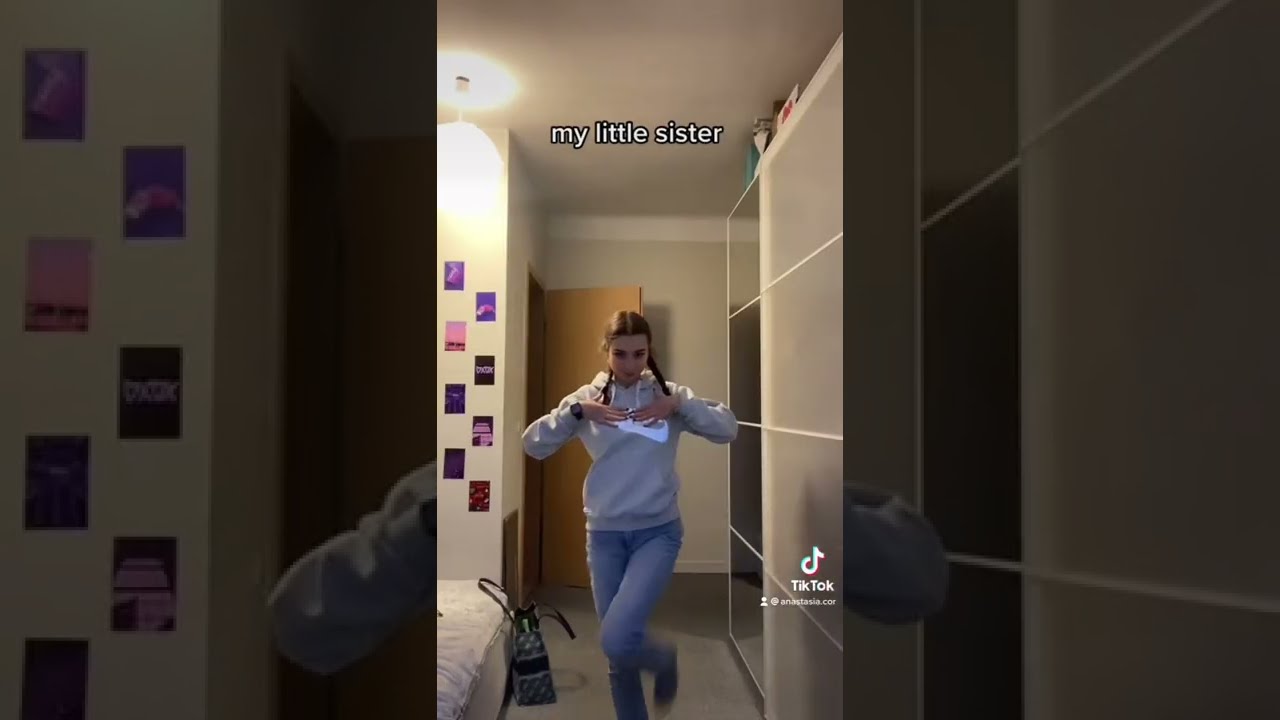The image is a multi-photo collage showing a girl in a small dorm room. The central picture, well-lit and detailed, features the girl who appears to be dancing, possibly for a TikTok video. She has brown hair, parted in the middle and styled in pigtails draping over her shoulders. She wears a gray hoodie with a white design, blue jeans, and her left knee is bent into the air while her hands rest on her chest. A brown door is visibly open in the background, and a bed is situated to her right with a black and white handbag on the floor. Above her, white text reads "my little sister," and a TikTok logo is seen in the lower right corner. The darker, zoomed-in flanking images highlight the background details: to her left are colorful postcards hanging on the wall, and to her right you can see a tiled wall. Both side images also capture segments of her room, including parts of her arm and the surrounding decor, providing a comprehensive view of the setting.